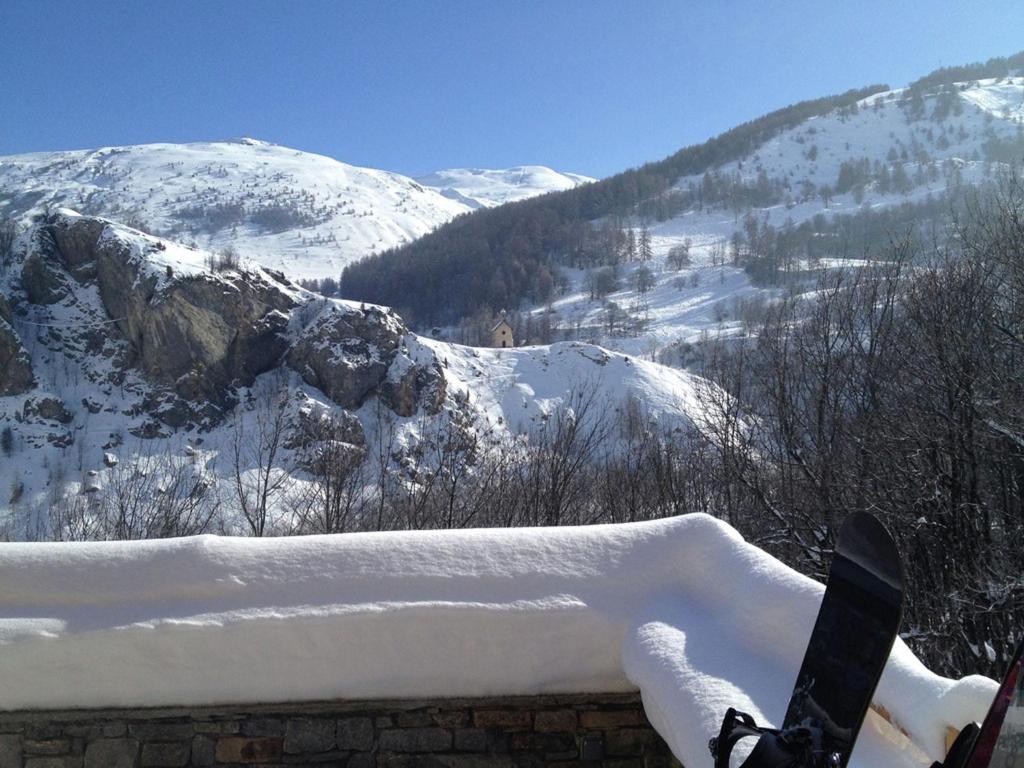The photograph captures a serene winter scene likely from a balcony or patio area in a mountainous ski resort. The ledge is blanketed with fresh snow, and skis are propped up against it, hinting at recent snowfall and imminent skiing activities. The landscape extends into snow-covered mountains, where rocky outcrops peek through the white, and trees—some bare and some dusted with snow—dot the slopes. Notably, there is scattered vegetation and small saplings in the vicinity. The background highlights rugged, snow-clad mountains under a brilliant, cloudless blue sky, enhancing the vivid snowy brightness. A building is also visible in the distance, further suggesting this could be someone's mountain home or part of the ski resort infrastructure. Overall, the clear blue sky and bright snow depict a crisp, clear day perfect for winter sports or enjoying the splendid natural beauty.